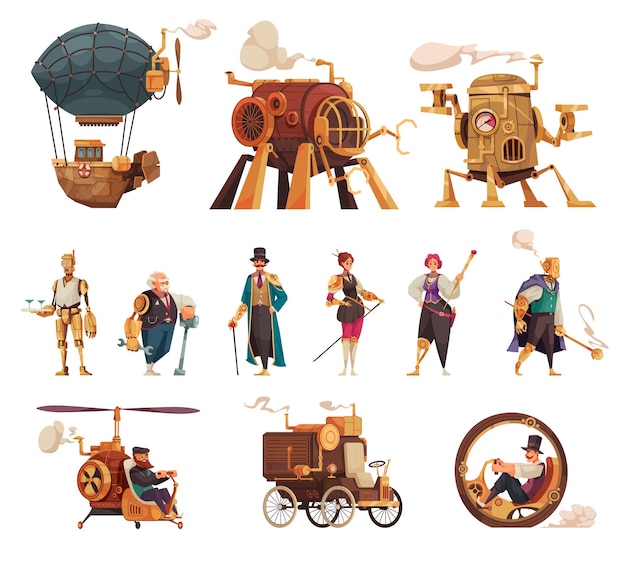The image is a steampunk-themed collection of various detailed illustrations arranged across three rows. 

**Top Row:** This includes three unique steampunk-inspired machines. The first is a dirigible with a dark bluish air balloon, complete with a boat and life preserver attached underneath. The second machine, positioned in the center, resembles a spider-like tank robot, intricately designed with mechanical legs. The third machine is a cylindrical, four-legged robot, noted for its temperature sensor and emitting smoke, with a gold-colored body reminiscent of R2-D2.

**Middle Row:** Here, six humanoid characters with cybernetic enhancements are depicted. They include a robotic individual carrying martinis, an old mechanic missing his right arm, a gentleman in a top hat with a cane, a lady wielding a long staff, a lady with a cane missing her right leg, and a gentleman holding a large scepter, missing his right leg and arm. 

**Bottom Row:** This row showcases three vehicles, each driven by different individuals. On the left is a single-person helicopter, in the middle is an unmanned car, and on the right is a single-wheeled car or bicycle.

This detailed arrangement beautifully captures the essence of the steampunk genre, blending advanced machinery with Victorian-era aesthetics.